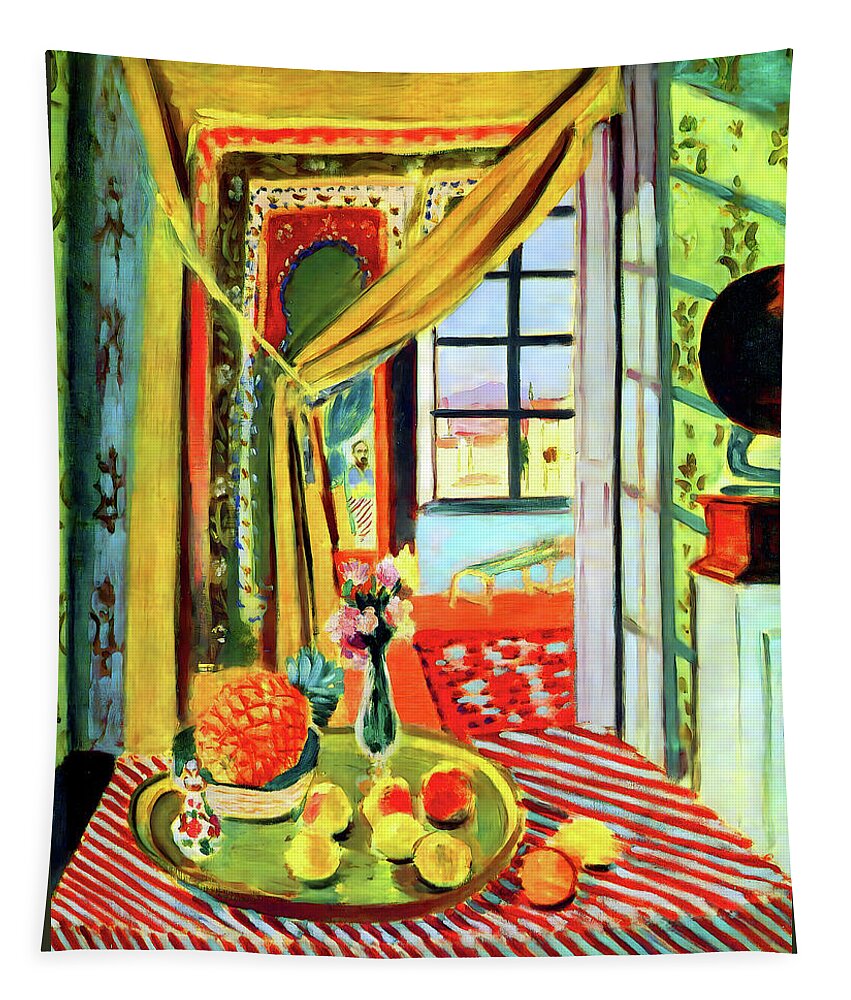The painting depicts a still life scene centered around a square table adorned with a red and white diagonally striped tablecloth. Atop the table rests a misshapen green plate holding approximately six oranges or peaches, with a couple of additional fruits placed outside the plate to the right. Also on the plate is a bowl containing a sideways pineapple, its stem and leaves extending towards the right. A small glass vase with a bouquet of yellow and pink flowers is situated to the right of the pineapple, while a small jar can be seen in front of the pineapple, slightly to the left.

Behind the table, a doorway features a yellow curtain tied back with a rope, revealing a hallway that leads to a room with red carpeting and a paned window offering a glimpse of a cityscape beyond. To the right of the table, resting on a shelf or cabinet, is an old phonograph, with its wooden base and part of the speaker visible.